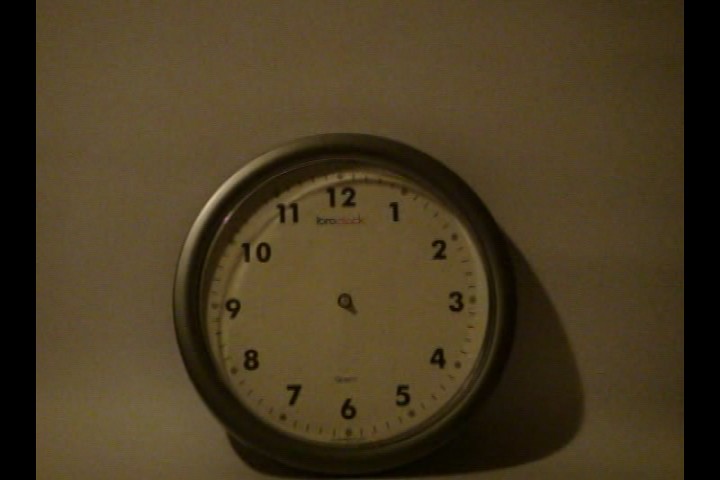This photograph captures a handless clock mounted on a white surface, likely an indoor wall. The lighting is dim, suggesting the photo was taken without a flash, with the primary light source in the upper left corner, casting a shadow of the clock down and to the right. The clock has a silver frame surrounding a white face, marked with standard black numerals from 1 to 12. Beneath the '12' is an unreadable brand name in a mix of black and red text, and the word "quartz" appears above the '6'. Along the sides of the white wall are dark lines, which could indicate either the edges of the wall or possibly screen artifacts from the original photo.